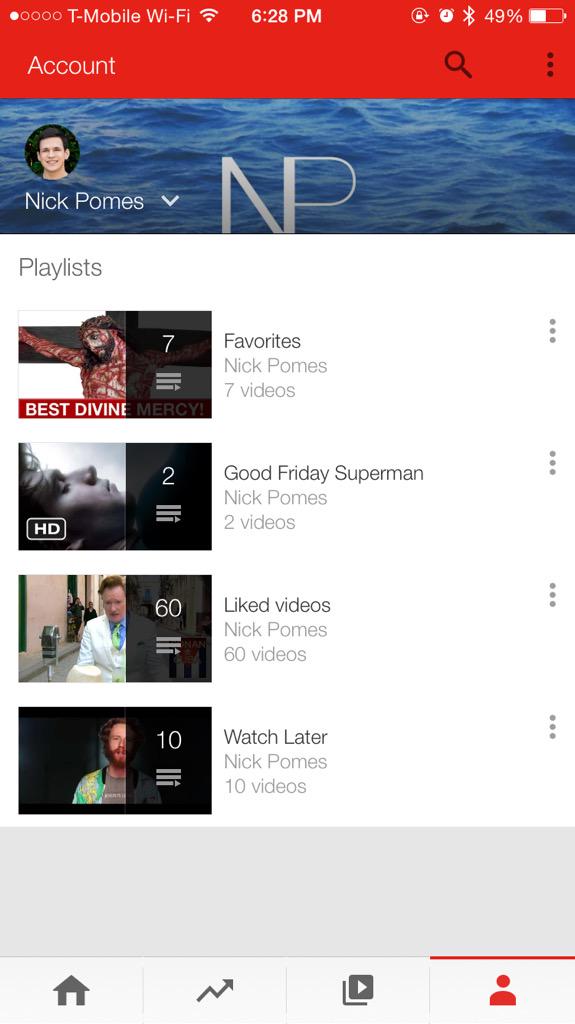This is a color image of a website interface designed for a mobile phone. At the top of the screen, there is a red header with white text displaying the network provider "T-Mobile," Wi-Fi status, and the current time, "6:28 pm," flanked by mobile icons on the right, including a battery icon indicating 48% charge.

Below the header, the left side of a navigation bar reads "Account," and the right side features a black search icon and an arrow icon. Underneath, a blue band resembling waves of water stretches across the screen. On the left side of this band, there is a small circular profile picture of a young man with light skin and dark hair, clean-shaven, and known as Nick Porneo. His name is displayed beneath the picture along with a grey "NP" monogram in the middle and a downward arrow beside his name.

The main section of the image shows a white background with grey text. The top left corner reads "Playlists," followed by four playlist thumbnail pictures. The first playlist, titled "Favourites," contains seven videos and has a small image that appears to depict Jesus on the cross. The second playlist, "Good Friday Superman," contains two videos and features a black-and-white image of a woman looking upwards. The third playlist, "Liked Videos," includes sixty videos and showcases a man in a white coat and blue shirt. The fourth playlist, "Watch Later," consists of ten videos and has a partial image of a man with a reddish beard wearing a blue and green shirt against a lighter background.

At the bottom of the screen is a grey rectangle with navigation icons. These icons, from left to right, include a black "Home" icon, an arrow icon, a YouTube icon, and a red "Person" icon on the far right.